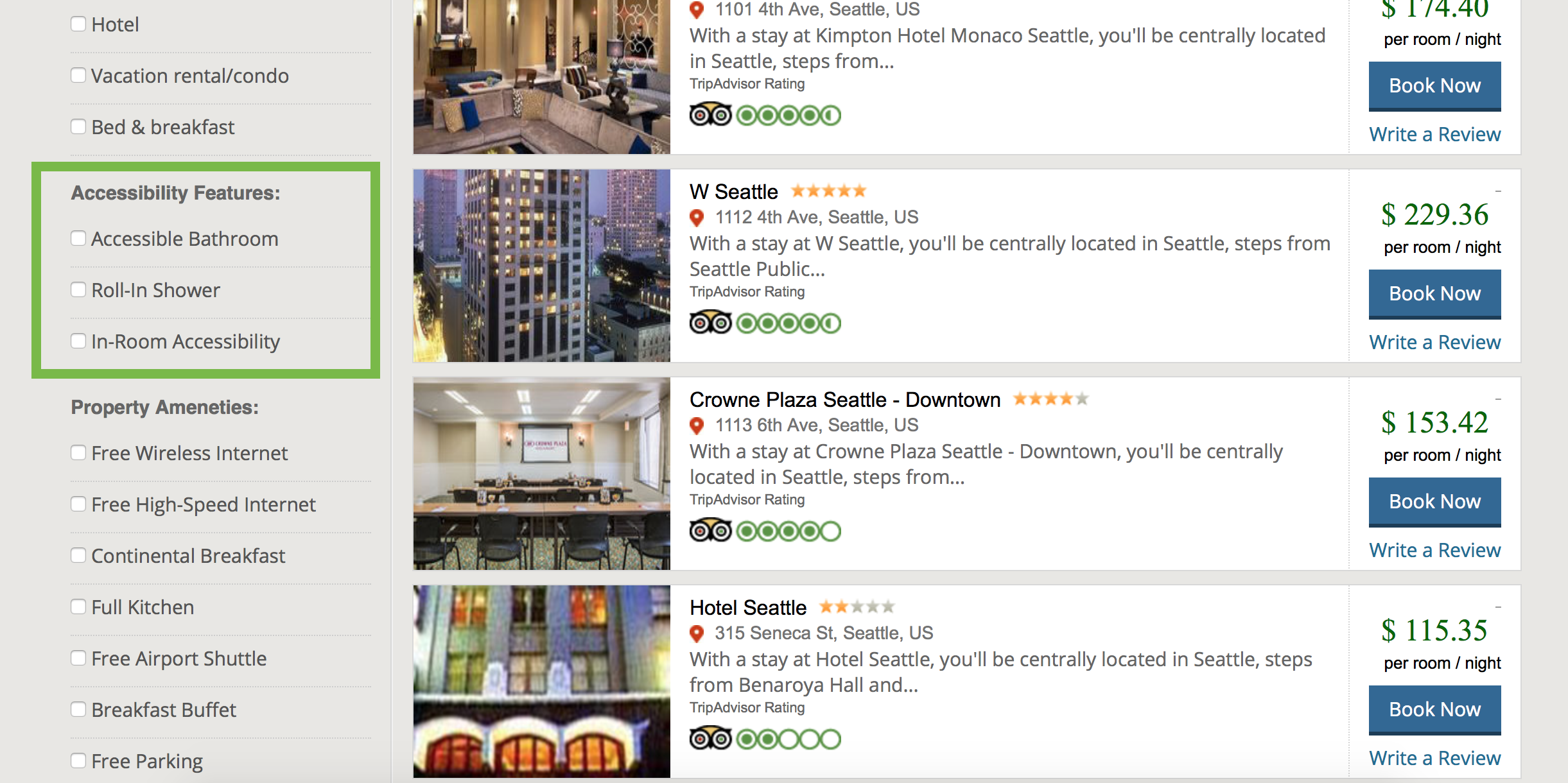This image is a screenshot taken from a TripAdvisor page, focusing on a section listing various accommodations. The left side of the image features a light gray sidebar menu with options to check different categories such as "Hotel," "Vacation Rental," "Condo," "Bed & Breakfast," and a variety of accessibility features like "Accessible Bathroom," "Roll-in Shower," and "In-Room Accessibility," all enclosed within a green-bordered box. 

Beneath that, property amenities are listed, including "Free Wireless Internet," "Free High-Speed Internet," "Continental Breakfast," "Full Kitchen," "Free Airport Shuttle," "Breakfast Bar," and "Free Parking."

The main section displays four listings, though the top listing is partially cut off, showing only a photo that appears to be from a lounge area and no other details.

The first complete listing is for "W Seattle," showcasing a high-rise building illuminated at night. This hotel has a perfect rating of five gold stars. Below it, the "Crowne Plaza Seattle Downtown" is featured, with a rating of four and a half gold stars and an image that seems to be from a conference room. The third listing is "Hotel Seattle," which has a lower rating of two gold stars and shows a photo of the building's exterior.

On the right side of each listing is a blue, rectangular "Book Now" button with white text, offering a quick and easy way to make a reservation.